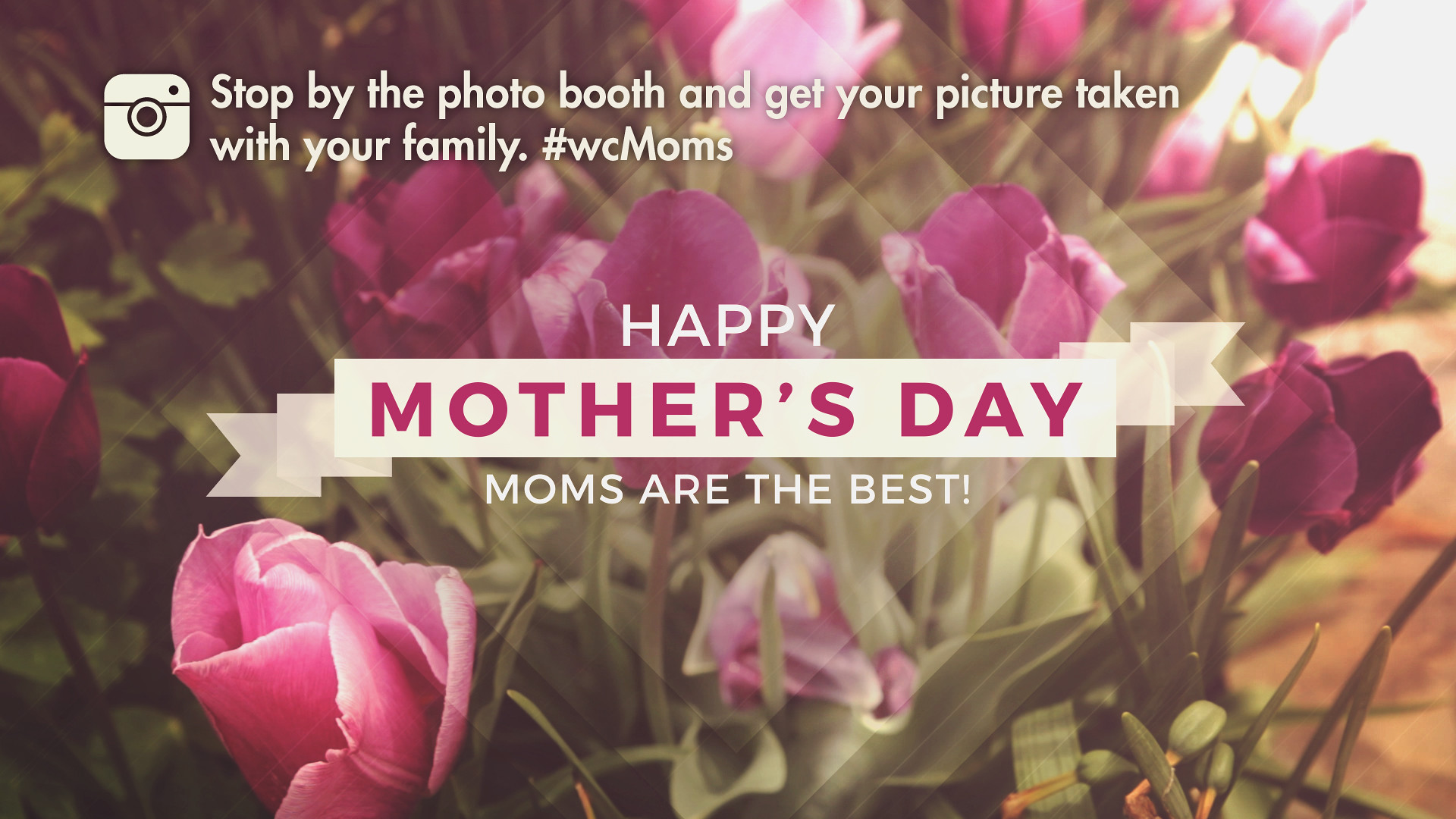The image is a visually appealing advertisement for Mother's Day with a background filled with vibrant green leaves and pink and purple flowers, possibly tulips or roses, set against what looks like an outdoor setting with some dirt visible on the right side. In the upper left corner, there is a design reminiscent of the Instagram app logo, featuring a square with a circle in the middle, a line to the top, and a small circle on the upper right side. Next to this is a message in white text that reads, "Stop by the photo booth and get your picture taken with your family," followed by the hashtag "#WCMoms." Below this message, a banner with a white background prominently displays the greeting "Happy Mother's Day" in purple text, with "Moms are the best" written in white underneath. The banner has a diamond-like shadow effect superimposed on the flowers. In the very upper right corner, there is a white flash glaring over one of the flowers, adding a touch of natural light to the scene. Overall, the advertisement creates a warm and inviting atmosphere, celebrating Mother's Day with colorful floral elements and inviting viewers to engage by taking family photos.